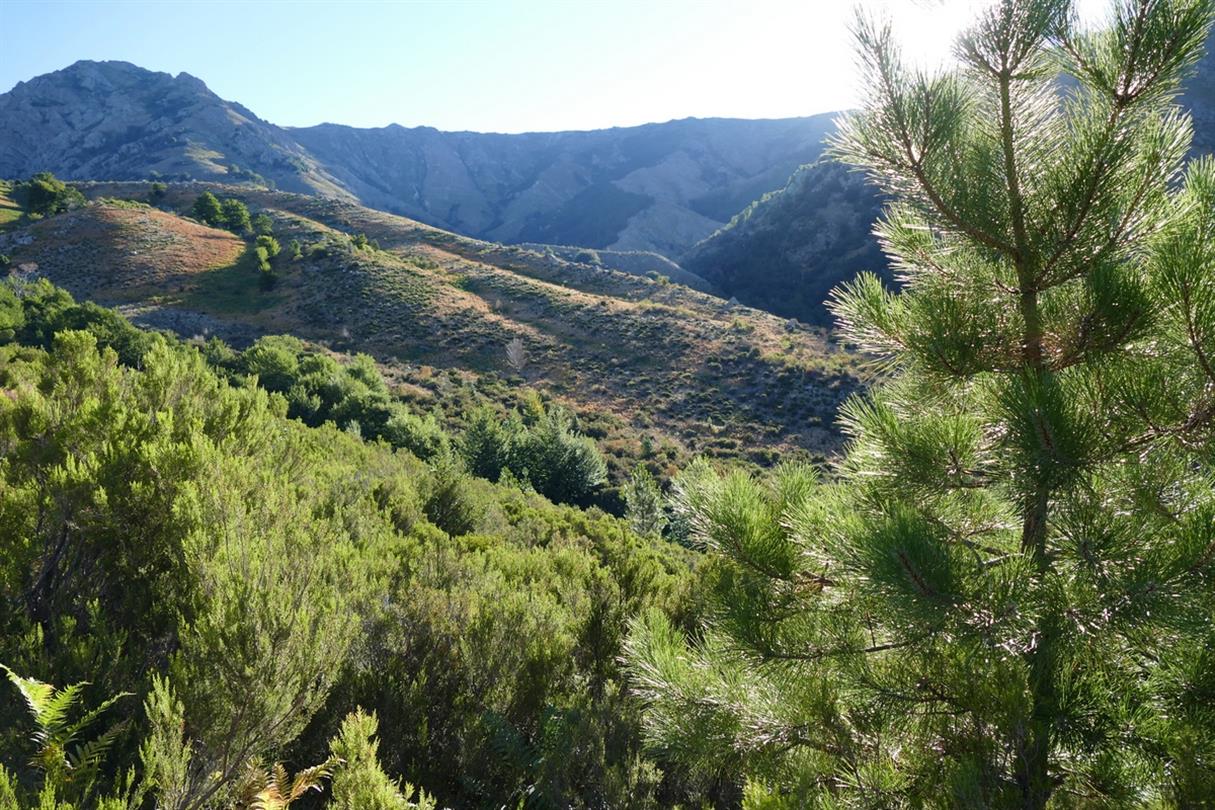This is a professionally taken landscape photograph depicting a sunlit, natural outdoor scene. The sky, which occupies a very thin strip at the top, transitions from light blue on the left to a whitish area partly obscured by a large, dark green pine tree on the right that visually dominates about a third of the image. The mountainous terrain in this image consists of rolling hills and distant mountains, covered with patches of bare rock interspersed with areas of dark green vegetation, including trees, shrubs, and grasses. The foreground features a mingling of rich green bushes and sparse, lighter green shrubs amidst brown, rocky ground. While the mountains present a mix of brown and gray hues, there’s also touches of yellowish-green foliage nearer the front. The overall composition is accentuated by the natural lighting, highlighting a variety of neutral shades with bursts of blue, yellow, and green, emphasizing the untouched beauty of the landscape. No people or animals are present, focusing solely on the serene and vibrant natural environment.